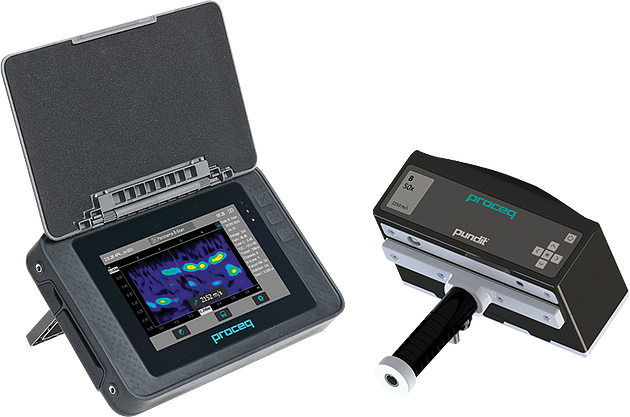The image depicts two pieces of electronic equipment manufactured by the company Proceq. The first device, positioned on the right, has a long rectangular shape with a black handle that appears to be made of foam. It features the word "Proceq" in turquoise and "pundit" in white, along with several directional arrows and a gray box labeled "B-F-I-T-T-X" and other smaller, indistinct text. This piece evokes a sense of vintage photography tools, though its exact function is unclear. The second device is a high-tech gadget with a screen that displays blue and thermal imaging. This device has a cover that flips open, revealing a display readout that can be positioned at an angle with the aid of its stand. The body of the gadget is in various shades of gray and black, and it also bears the company name "Proceq" in turquoise lettering. Both devices are sophisticated and seem integrated for specific technological applications, though their precise uses are not entirely clear.